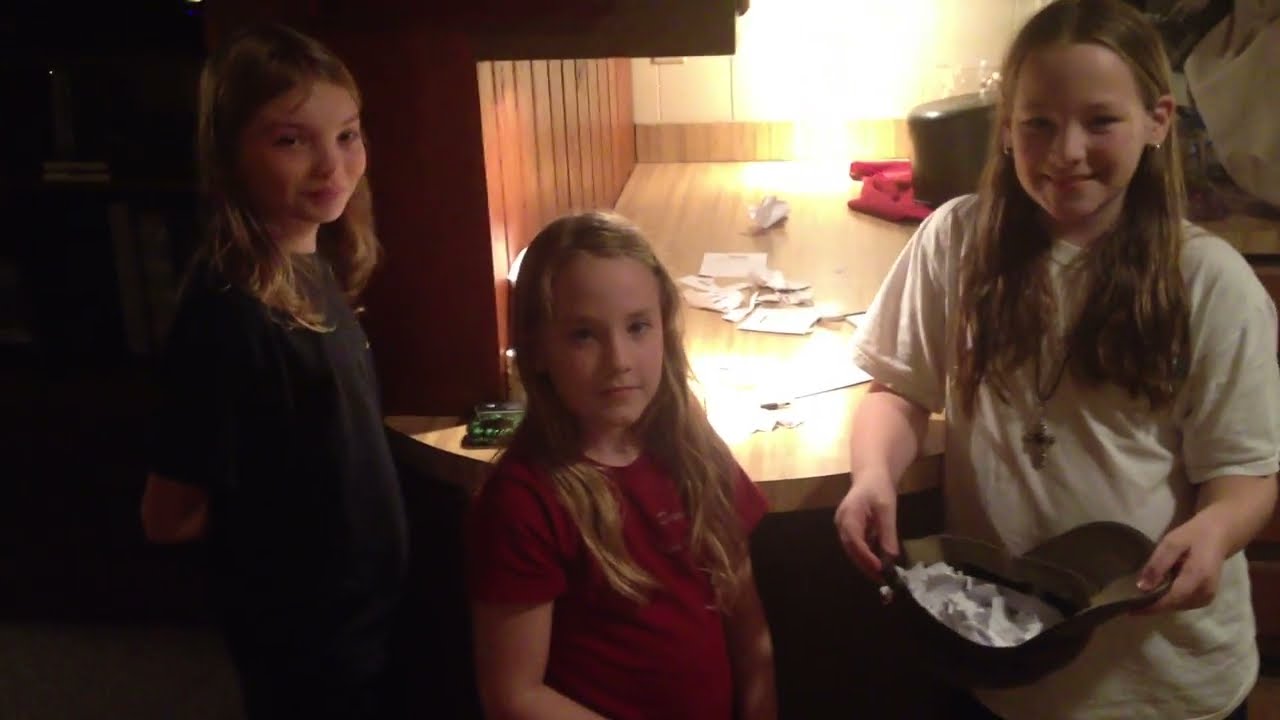In this image, we see a young girl, around eight or nine years old, standing at the center and holding an upside-down baseball cap filled with crumpled pieces of paper, seemingly for a pick-something-out-of-a-hat game. She has long brown hair cascading over her shoulders and is dressed in a loose-fitting white t-shirt, adorned with a silver cross necklace. To her left, partially visible, is another girl with long blonde hair, covering her eyes with a gloved hand, adding an element of surprise to the game. The background reveals a kitchen setting with countertops cluttered with various items including torn pieces of paper, a box, and bananas. An assortment of objects, including a sink and soap, can also be seen, placing the scene firmly in a domestic environment.